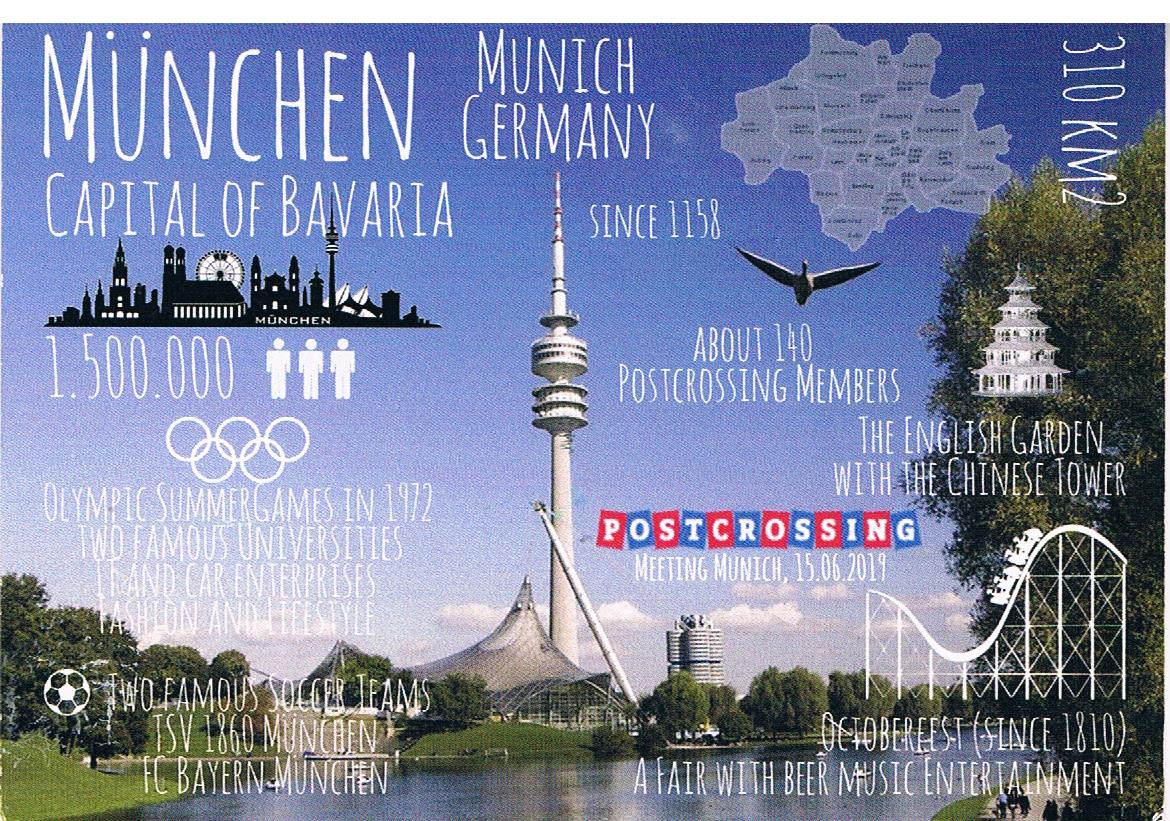This image is a detailed poster of Munich, Germany, set against a blue background filled with text and images. The central feature is a tall, thin needle-shaped tower, possibly the Olympiaturm, with a small dome-like tent structure beneath it. To the right of the tower, there is an illustration of a roller coaster symbolizing the Oktoberfest, noted for beer, music, and entertainment, held since 1810. The top text reads "München, capital of Bavaria," emphasizing its rich heritage and large population of approximately 1.5 million.

Below the tower text indicates notable points such as the hosting of the 1972 Olympic Summer Games, iconic landmarks like the English Garden and the Chinese Tower, and notable institutions like two famous universities. Additionally, it highlights Munich's automotive enterprises, fashion, and lifestyle.

Lower sections mention two prominent soccer teams—TSV 1860 München and FC Bayern München. A map of Munich is present, with text marking the city's founding year as 1158 and noting about 140 Postcrossing members. Also depicted are the five interlinked Olympic rings and icons representing people, underscoring the city's vibrant community and historic events. The image offers a panoramic view of the cityscape, with a river or lake in the foreground under a bright sky, making it an informative and visually engaging depiction of Munich.